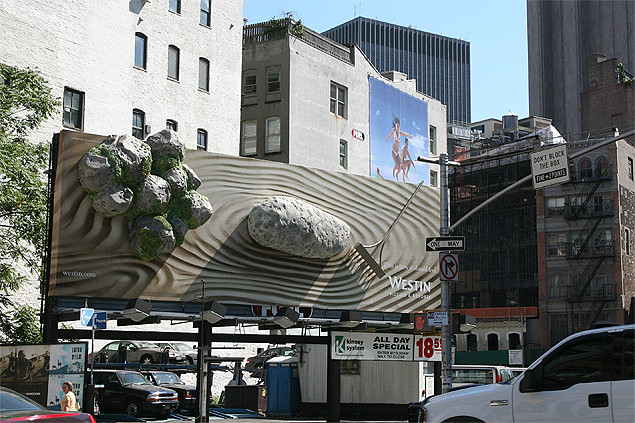In this rectangular image, we observe an urban scene from a slightly elevated viewpoint, as though the picture was taken from the side. The sky is a simple, light blue expanse with no visible clouds or dimension, creating a serene backdrop. The cityscape is dominated by tall buildings and gray blocks with a tan, stone beige hue, punctuated by various billboards.

In the foreground, close to a light pole equipped with a traffic light, a dilapidated building stands out. To the bottom right of the image, a white truck or car is parked. A significant billboard reading "Weston" commands attention with its three-dimensional design, featuring large, gray rocks that appear to be bursting out. This billboard is positioned in the upper left quadrant of the image, with the rocks varying in size and literally popping off the billboard. Below it, the sign advertises an "All Day Special 1859."

Additionally, more cars are parked in a nearby parking lot, and a solitary tree stands to the left, adding a touch of nature to the otherwise urban setting.